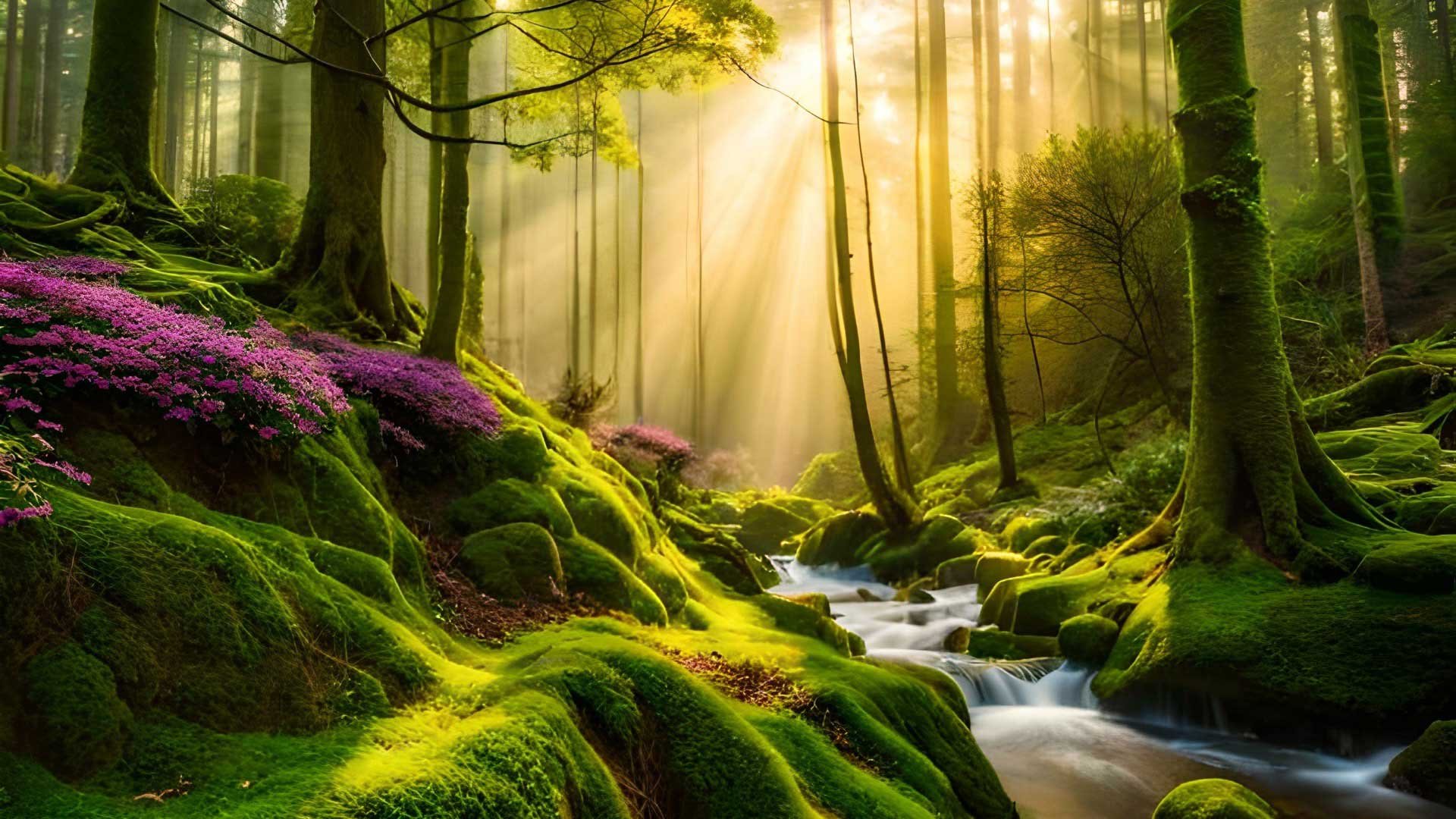This AI-rendered painting depicts a serene forest scene, centered around a gently babbling creek with soft white water cascading over several levels, culminating in a tranquil brown water section at the bottom left. The creek is flanked by verdant, moss-covered rocks, which are illuminated by rays of sunlight filtering through the dense canopy above, creating a patchwork of light and shadow across the scene. On the right, a robust tree trunk, its bark entirely shrouded in green moss, stands tall amidst the lush undergrowth of equally mossy ground. The left side features a steep, moss-laden bank that levels off before ascending again, where clusters of tiny purple flowers add a splash of color to the greenery. The background is filled with more tree trunks, some bearing branches adorned with pine needles, adding to the dense, wooded atmosphere. Beams of soft, diffused yellow light penetrate the forest, lending the entire scene a magical, almost fantasy-like quality reminiscent of Tolkien's enchanted forests.